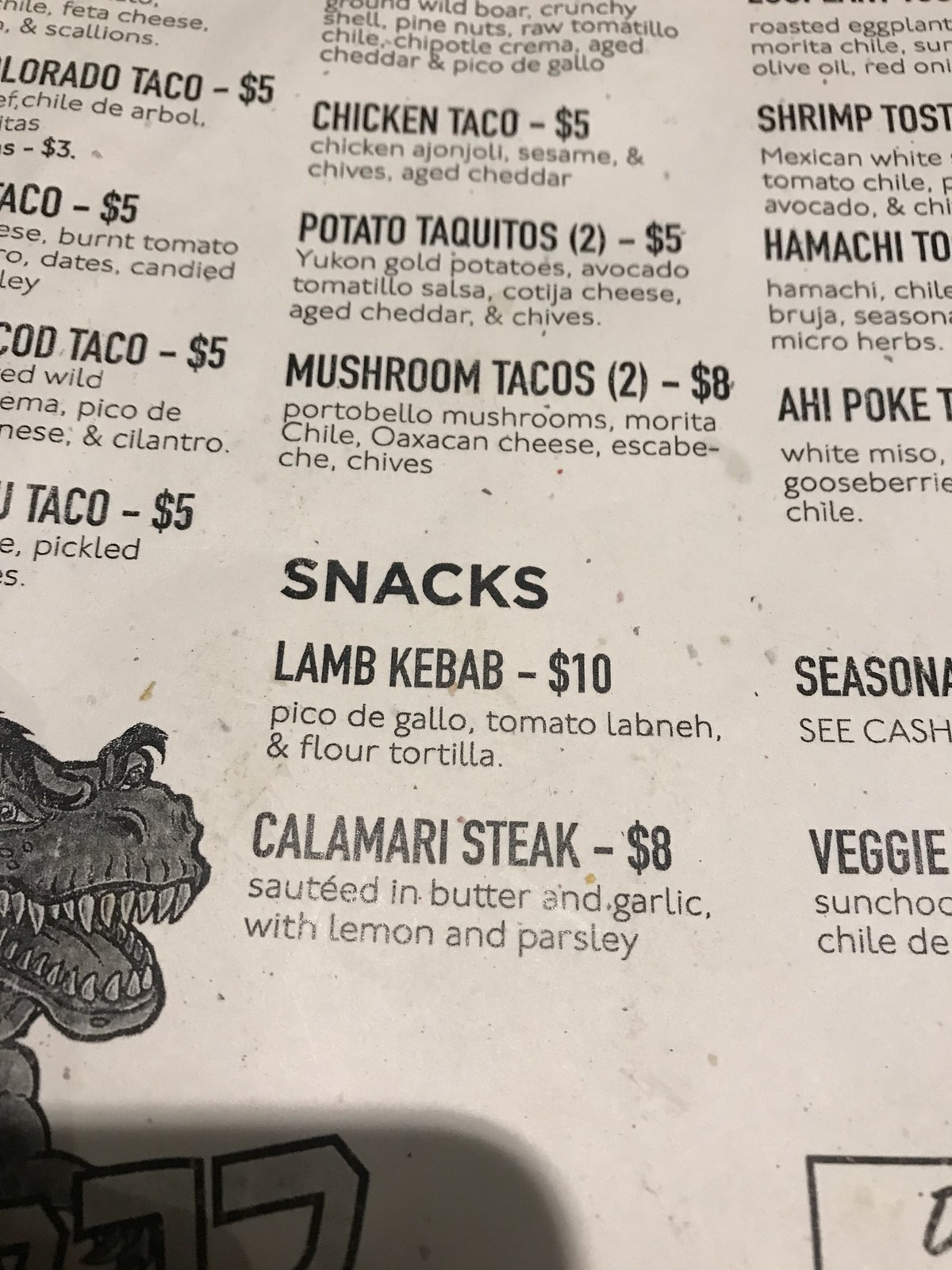The image depicts a section of a menu with three columns of items, primarily featuring tacos and snacks. In the bottom left corner, there is a detailed drawing of a dragon with its mouth open, displaying sharp teeth on both the top and bottom jaws. The dragon also has prominent eyebrows with hair and is illustrated in a vivid artistic style.

The first column lists several taco options, each priced at $5:
- Lorado Taco
- Taco
- Cod Taco
- Another taco listing with unspecified details but priced at $5, accompanied by pickles.
- Chicken Taco described with ingredients such as chicken a jornoli, sesame, chives, and aged cheddar.

The menu also includes:
- Potato Taquitos for $2
- Mushroom Tacos for $5

Underneath these items, there is a section titled "Snacks" that includes:
- Lamb Kebab for $10, served with pico de gallo, tomato labana, and flour tortilla
- Calamari Steak for $8, sauteed in butter and garlic with a hint of lemon

A third column is present on the right side of the image, although its contents are not entirely visible in the picture. Each section of the menu has varying text shades, with some items written in a darker shade and others in a lighter, less legible shade.